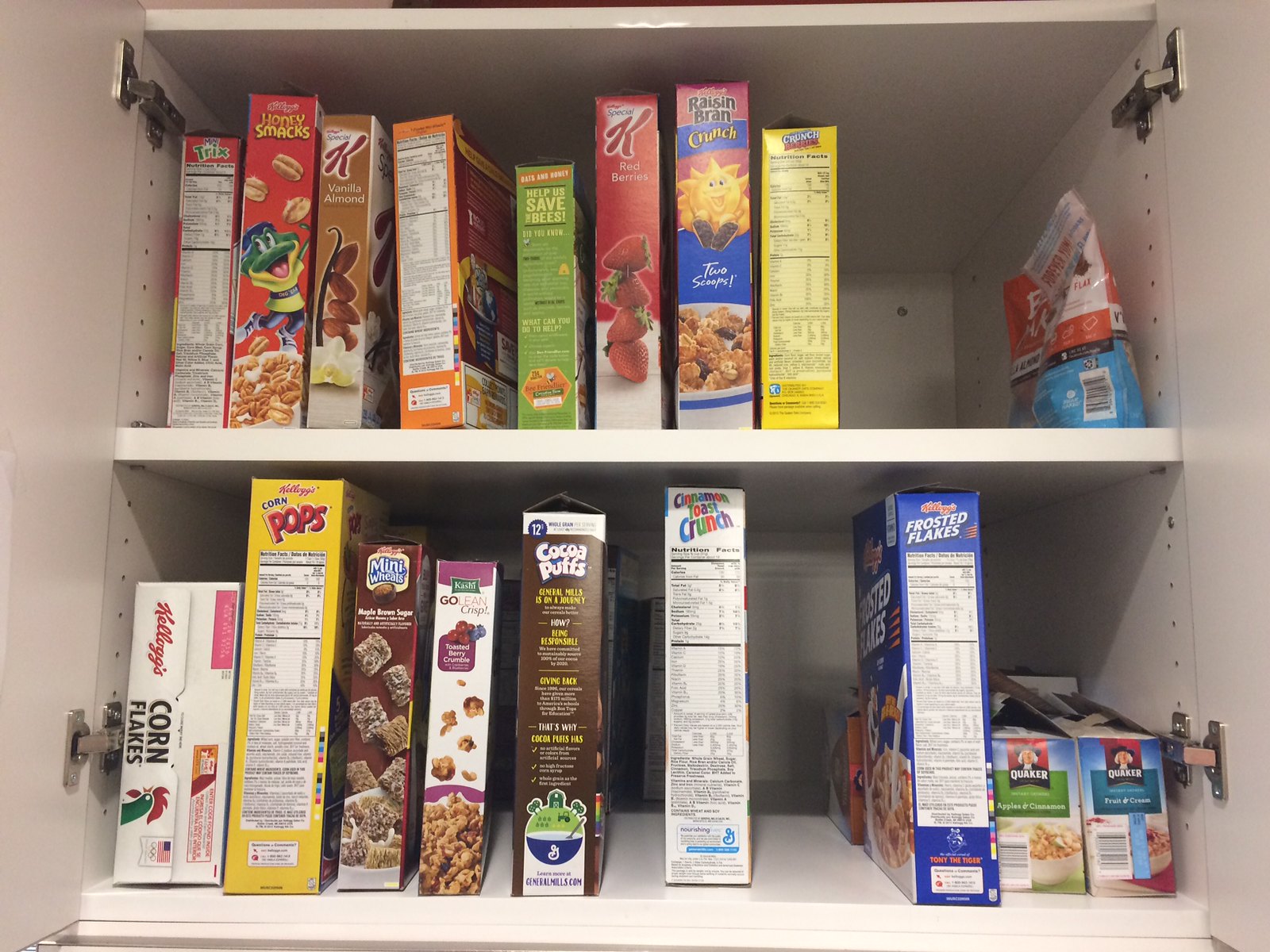This image depicts a neatly confined kitchen cabinet with its white double doors open, revealing two shelves filled with a variety of breakfast cereals. The cabinet's interior is a basic off-white color, and the silver hinges are visible on either side of the doors. The bottom shelf is densely packed with seven different boxes of cereal, including Frosted Flakes, Cinnamon Toast Crunch, Cocoa Puffs, Mini Wheats, Kashi, Corn Pops, and Corn Flakes. Additionally, this shelf holds two Quaker Instant Oatmeal boxes labeled Apples and Cinnamon, and Fruit and Cream.

On the top shelf, there are several more cereal boxes and a plastic bag containing granola. The cereals on this shelf include Trix, Honey Smacks, Special K Vanilla Almond, an unidentified box with an orange label, a smaller green box promoting bee conservation (possibly granola), Special K Red Berries, and Raisin Bran Crunch. There's also a Crunch Berry box in yellow and, on the far right side, the plastic bag of granola. The detailed arrangement and variety of cereals, combined with the visible text on the boxes, suggest this cabinet is specifically designated as the breakfast cupboard in someone's kitchen. There are no people visible in the image.